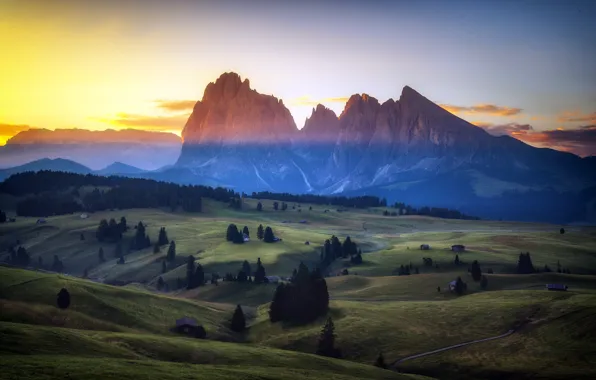The image is a full-color, square composition capturing the serene beauty of an outdoor landscape, likely during either sunrise or sunset. The upper left-hand corner of the image glows with the soft yellow hues of the sun, casting a gentle light onto scattered clouds which, towards the upper right, shift to darker tones. Below this sky, a majestic mountain range stretches horizontally, its rugged peaks dusted with a suggestion of snow and enveloped in a delicate blue haze at its base.

Descending from the mountains, the terrain transitions into a lush, verdant expanse dotted with numerous evergreen trees, their dark silhouettes standing in stark contrast to the vibrant green fields. The landscape is meticulously groomed, suggesting areas of mowed grass, perhaps indicative of farmland or well-maintained lawns. Among this greenery, there appear to be several small homes; one is particularly noticeable to the right, accessible via a small road in the lower right-hand corner of the image.

Overall, the scene's composition—from the glowing sky and majestic mountains to the verdant fields and scattered homes—exudes a tranquil, almost idyllic rural charm, perfectly encapsulating the harmonious interplay of natural elements under the gentle embrace of the setting or rising sun.